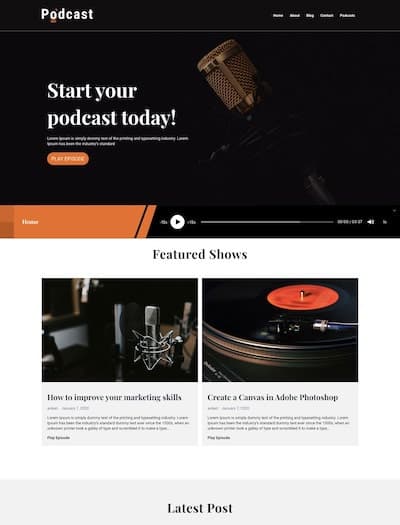Screenshot Description:

The screenshot captures a section of a website with a focus on podcasts. The top section features a black background with the word "Podcast" displayed in white text at the top left corner. The top navigation bar, also set against the black background, hosts five white links on its right side. A thin white line runs below the navigation bar, separating it from the main content.

In the main section, on the left side, there's a large tagline in white letters stating "Start Your Podcast Today." Below this tagline, a pill-shaped orange button invites users to take action. To the right of the tagline, there is an image of a brown microphone with a brown wire mesh top.

Directly beneath the orange button, an audio player is displayed. It features a circular white play button, with an orange section on the left and a black section on the right.

Further down, the section titled "Featured Shows" highlights two article images, offering a preview of the content available.

This detailed layout emphasizes the website's theme and invites visitors to engage with the podcasting content and tools available.